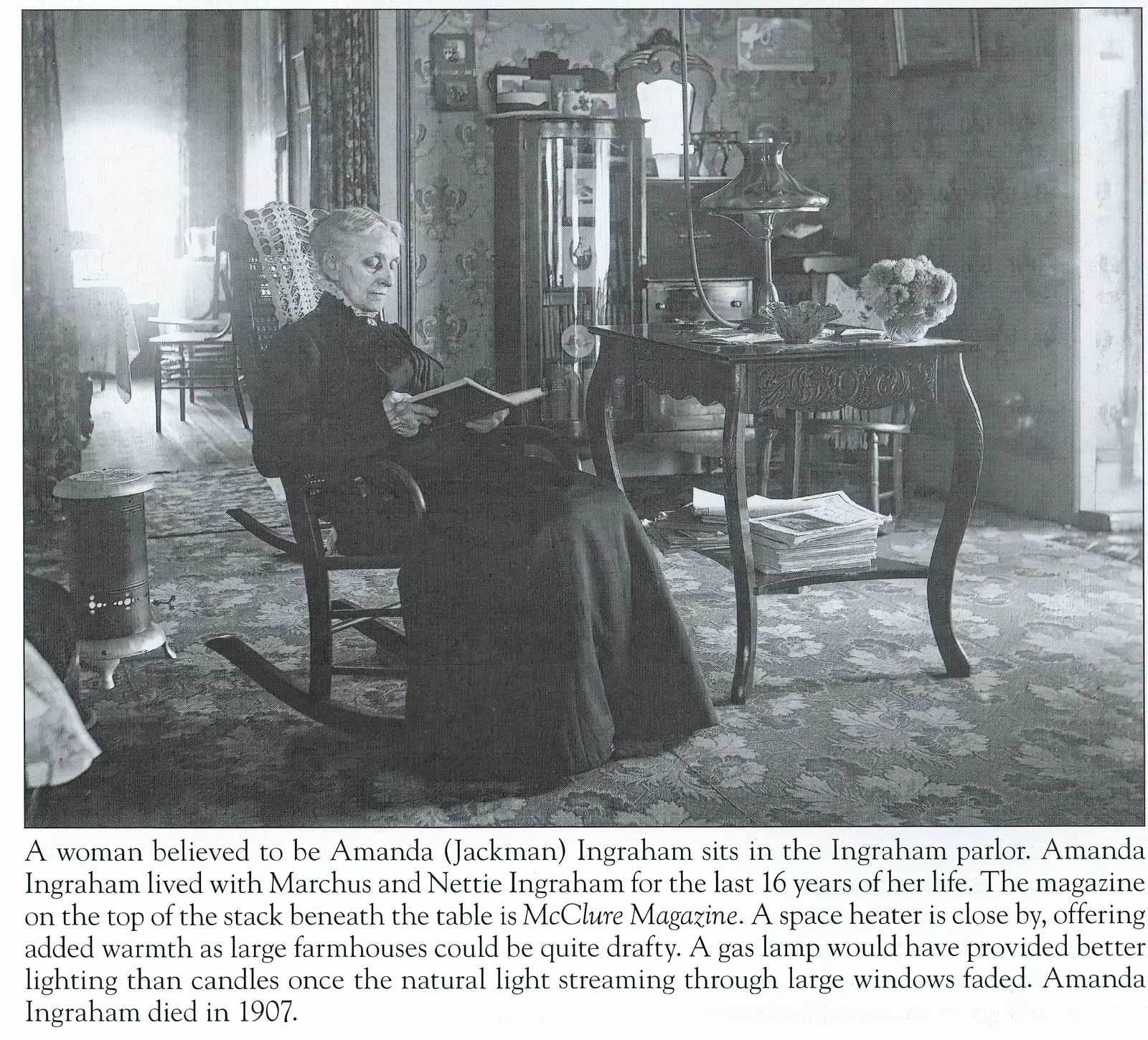In this black-and-white photograph, an elderly woman, believed to be Amanda Jackman Ingram, is seated in a wooden rocking chair. Her gray hair is neatly parted in the center as she concentrates on a book held in both hands. She is dressed in a long, black dress and her gaze is fixed on the open pages of the book. Positioned behind her on the right side is a holy white blanket, which adds a touch of warmth to the scene.

The room, likely the Ingram parlor, is furnished in an antiquated style that denotes the early 1900s. A wooden antique table sits to her side, topped with a lamp and a stack of papers, with McClure Magazine visible on top. A mirror adorns the wall behind the table, reflecting the room's modest decor.

The floor is covered with a gray carpet embellished with floral patterns, adding an element of coziness to the drafty farmhouse setting. A space heater is placed nearby for additional warmth, evidencing the need for heating in such large, airy homes. The black text on the white background beneath the image reads, "A woman believed to be Amanda Jackman Ingram sits in the Ingram parlor. Amanda had been engraved, lived with Marcus and Nettle Ingram for the last 16 years of her life. The magazine on top of the stack beneath the table is McClure Magazine. A space heater is close by offering added warmth. As large farmhouses could be quite drafty, a gas lamp would have provided better lighting than candles once the natural light streaming through large windows faded. Amanda Ingram died in 1907."